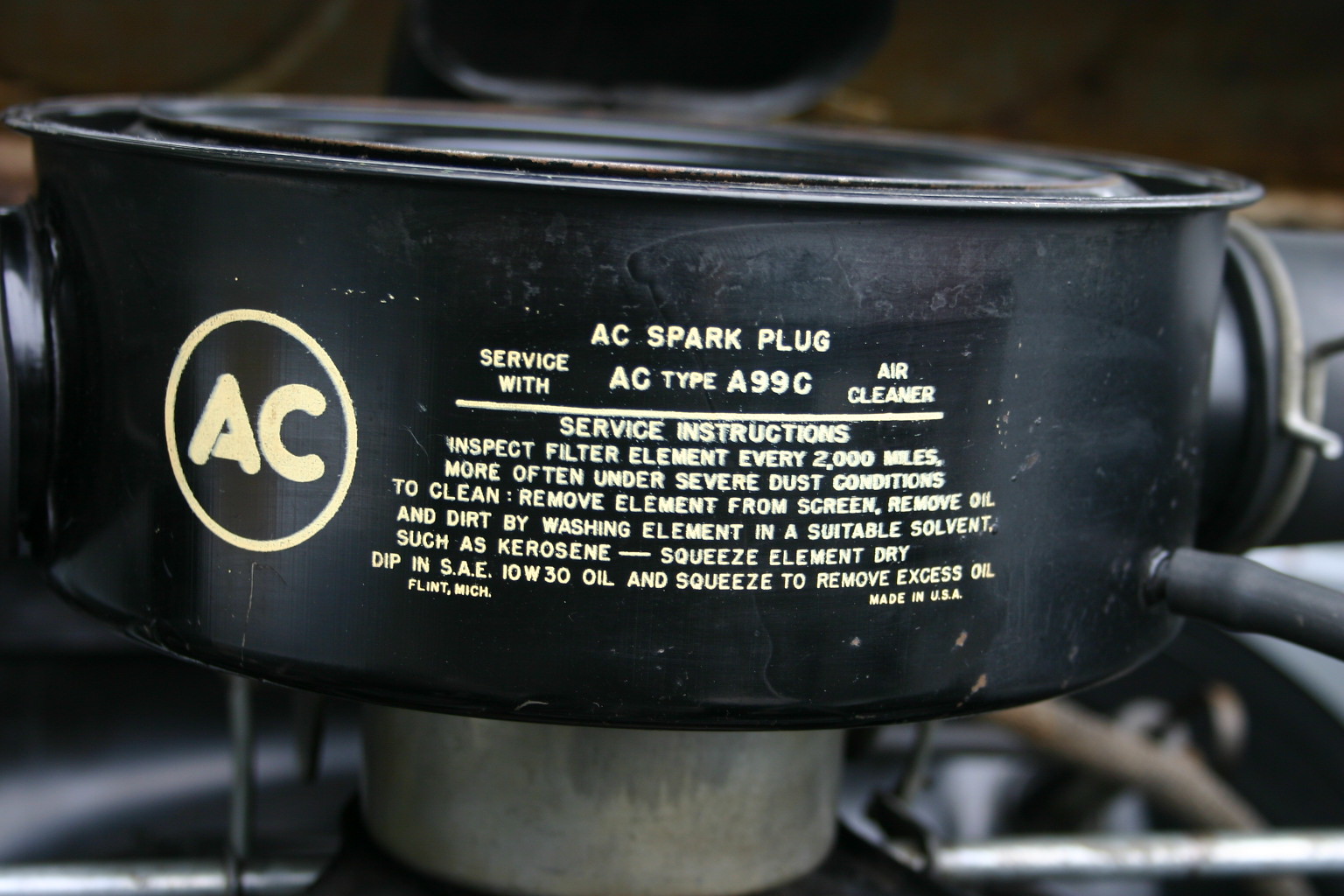The image features a close-up view of an AC spark plug component situated in what appears to be a factory or garage setting. Dominating the image is a black cylinder with a smaller silver cylinder beneath it. To the right of this component, there is a wire, and to the left, encircled in white, are the large, white capital letters "AC." Beside this, in large capital letters, it reads "AC SPARK PLUG," followed by "SERVICE WITH AC TYPE A99C AIR CLEANER" underneath.

A line separates this text from the service instructions, which are prominently displayed in white capitals and small letters: 
- "INSPECT FILTER ELEMENT EVERY 2,000 MILES, MORE OFTEN UNDER SEVERE DUST CONDITIONS."
- "TO CLEAN: REMOVE ELEMENT FROM SCREEN. REMOVE OIL AND DIRT BY WASHING ELEMENT IN A SUITABLE SOLVENT SUCH AS KEROSENE. SQUEEZE ELEMENT DRY. DIP IN SAE 10W30 OIL AND SQUEEZE TO REMOVE EXCESS OIL."

Finally, in small capitals below, it states "FLINT, MICHIGAN," and "MADE IN USA." The image, measuring approximately 8 inches wide by 6 inches tall, focuses sharply on the text and the spark plug, leaving the background slightly blurry to emphasize the instructional details and the part's branding.